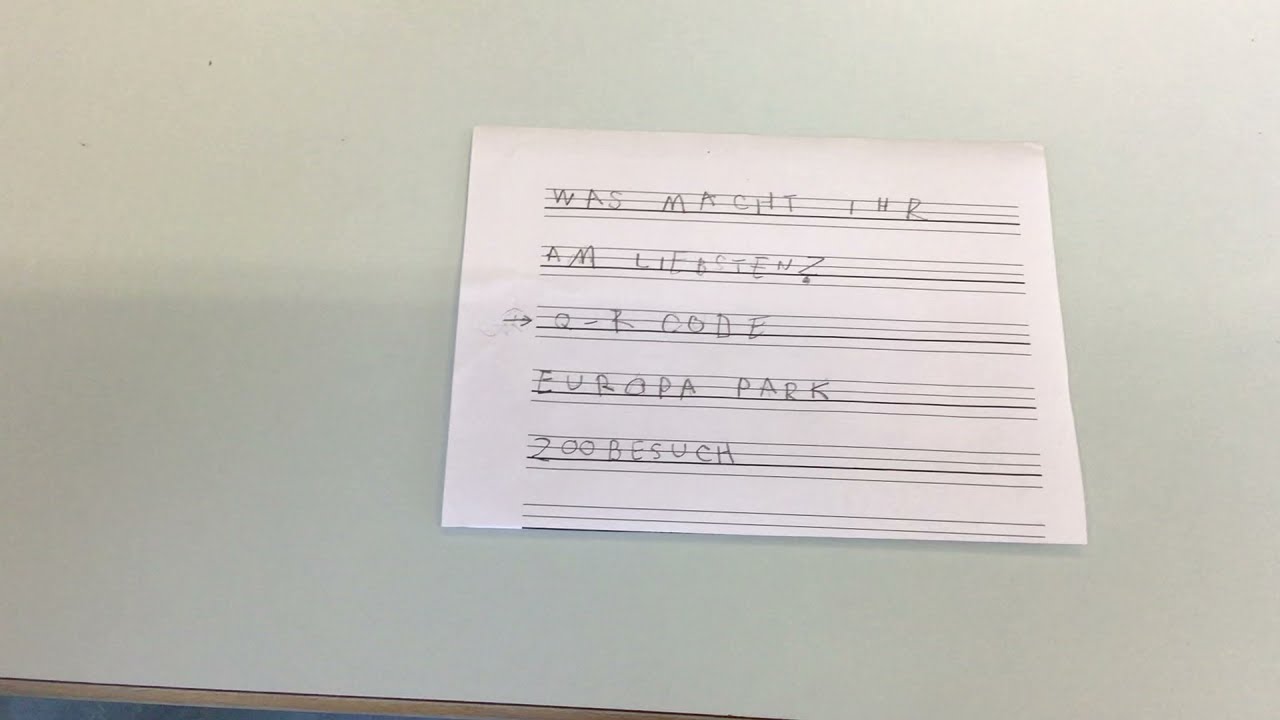The image shows a close-up of a piece of paper, placed on a white table, featuring a music log sheet with five distinct rows. Each row comprises four horizontal black lines, and a series of words written in capital letters in black ink. The words appear to be in a foreign language and are arranged as follows: the top row reads "WAS MACHT TNR," the second row "AMLIE BTEHZ," the third row "QIBOODE," the fourth row "AURPARK," and the fifth row "ZOOBESUZH". The paper is the focal point of the photograph, which is set against a simple backdrop of a white table and what appears to be gray flooring beneath the table.